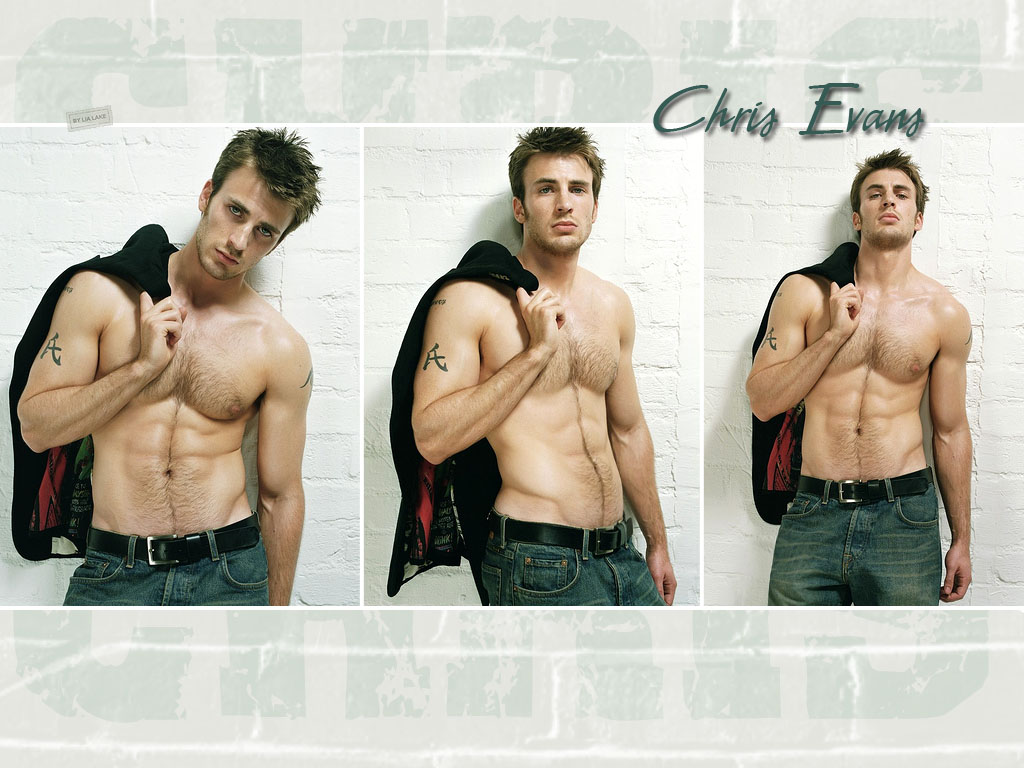This image series features three photos of Chris Evans, each with green text above that spells out his name, casting a subtle shadow. All three images capture him shirtless, wearing blue jeans with a black belt, and holding a black sweater draped over his right shoulder by his index finger. The setting appears to be a photo shoot against a white brick wall.

In the first photo on the left, Chris Evans is facing the camera directly, with his head tilted slightly to the left. The middle photo shows him in a profile view, his torso turned partially to the side, while he continues to look straight at the camera. In the final photo on the right, he stands straight again, his head tilted back as if looking down at the viewer, maintaining eye contact with the camera in each shot. The sequence captures a dynamic range of poses emphasizing his relaxed yet intense demeanor.